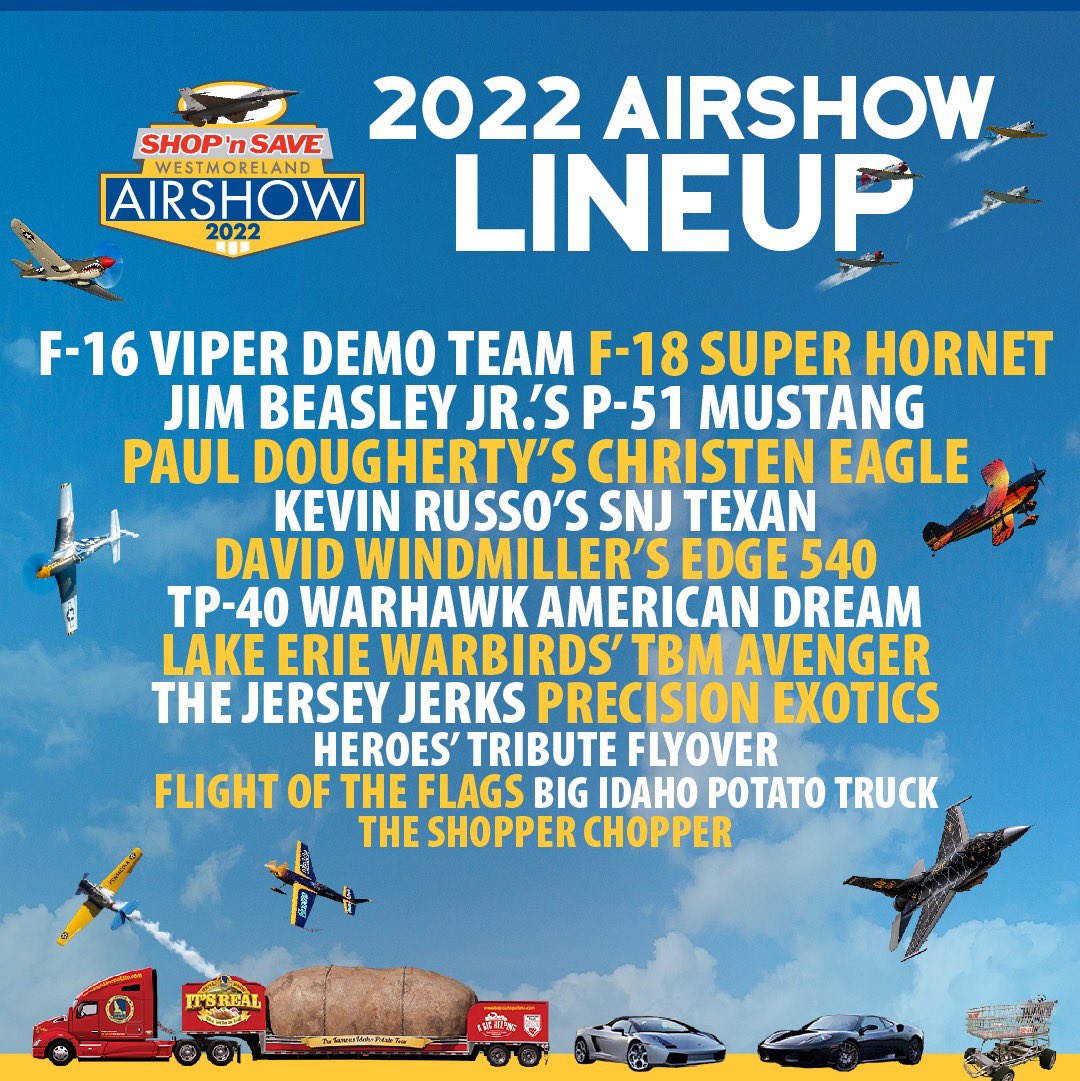This advertisement portrays the "2022 Westmoreland Airshow" with a vibrant sky-blue background accentuated by white, fluffy clouds. Dominating the right side, large white text reads "2022 Airshow Lineup," accompanied by several miniature airplanes flying in formation nearby. On the left side, a medallion features an airplane enclosed in a white circle, above red text reading "Shop and Save." Underneath, "Westmoreland" is displayed in dark text on a yellow background, followed by "Airshow" in white text against a blue background, and finally "2022" in blue text on yellow.

A detailed list of prominent participants includes: F-16 Viper Demo Team, F-18 Super Hornet, Jim Beasley Jr.'s P-51 Mustang, Paul Doherty's Christian Eagle, Kevin Russo's SNJ Texan, David Windmiller's Edge 540, TP-40 Warhawk American Dream, Lake Erie Warbirds' TBM Avenger, Jersey Jerks' Precision Exotics, Hero's Tribute Flyover, Flight of the Flags, Big Idaho Potato Truck, and the Shopper Chopper.

At the bottom of the image, a large red semi-truck is prominently featured carrying an enormous potato, flanked by two sports cars and a shopping cart. Various types of aircraft, including a noticeable red and orange plane and a military jet, are scattered throughout the scene, enhancing the dynamic and lively depiction of the airshow event.